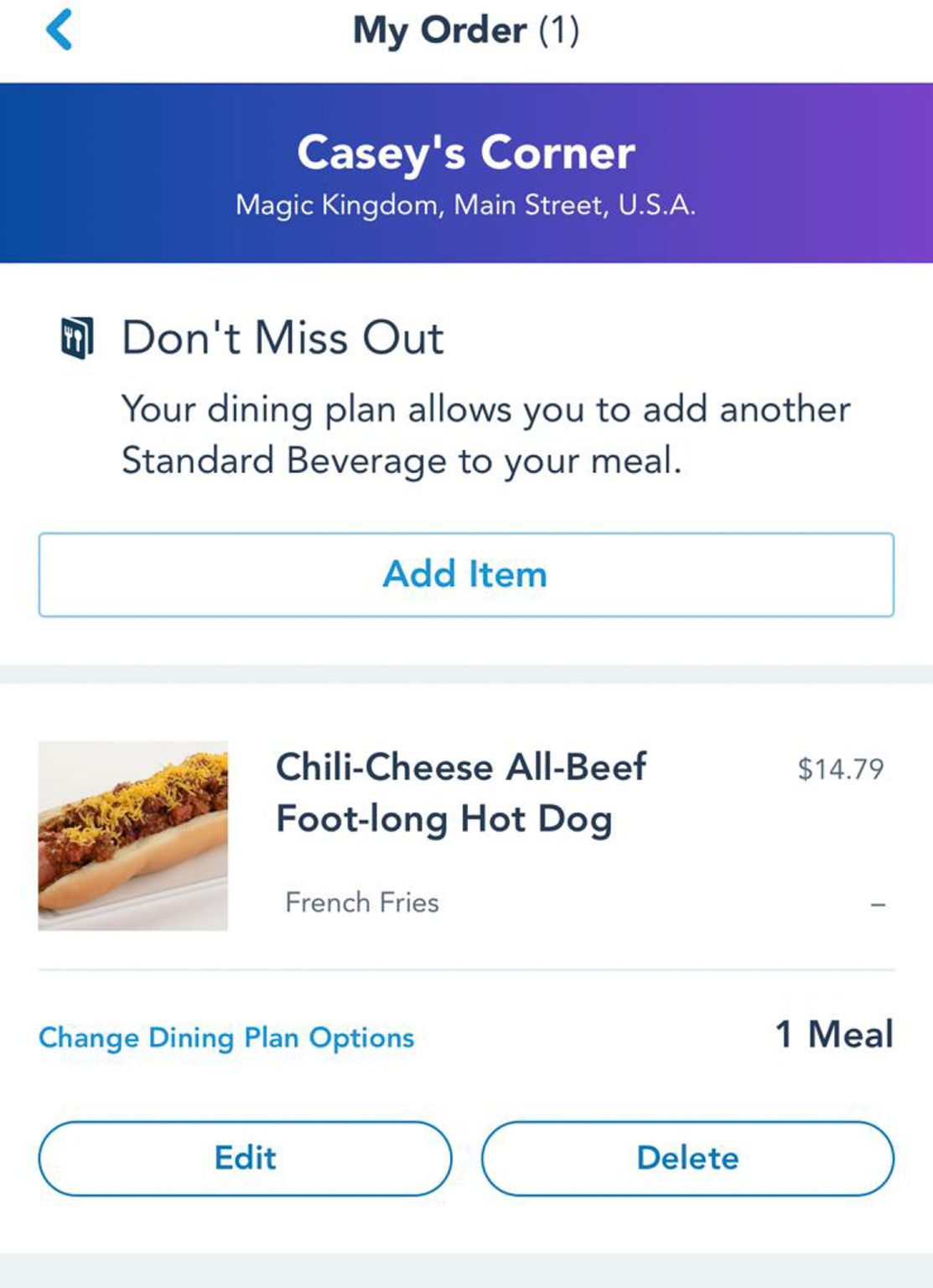The image depicts a digital ordering interface on a white background. At the top, a navigation bar with a back arrow is visible. Centered within this bar is the text "My Order (1)" in bold black font, with the number "1" in parentheses and not bolded.

Below this, a bluish-purple banner prominently displays "Casey's Corner" in bold white font, centered at the top. Just beneath this, in smaller, non-bolded white text, it reads "Magic Kingdom, Main Street USA," indicating that the location is at Disney.

Further down, there is an icon depicting silverware, accompanied by the text "Don't miss out" in black lettering. Below this, in smaller text, it states "Your dining plan allows you to add another standard beverage to your meal," informing the user of an available dining plan benefit.

An "Add Item" bar follows, leading to the detailed order summary. The order includes a "Chili Cheese All-Beef Footlong Hot Dog and Fries," priced at $14.79. The fries are mentioned to be complimentary. The interface allows options to change the dining plan, edit, or delete the item from the order.

The caption notes the high price of the meal, concluding with a remark, "Hope you enjoy that $15 hot dog and fries."